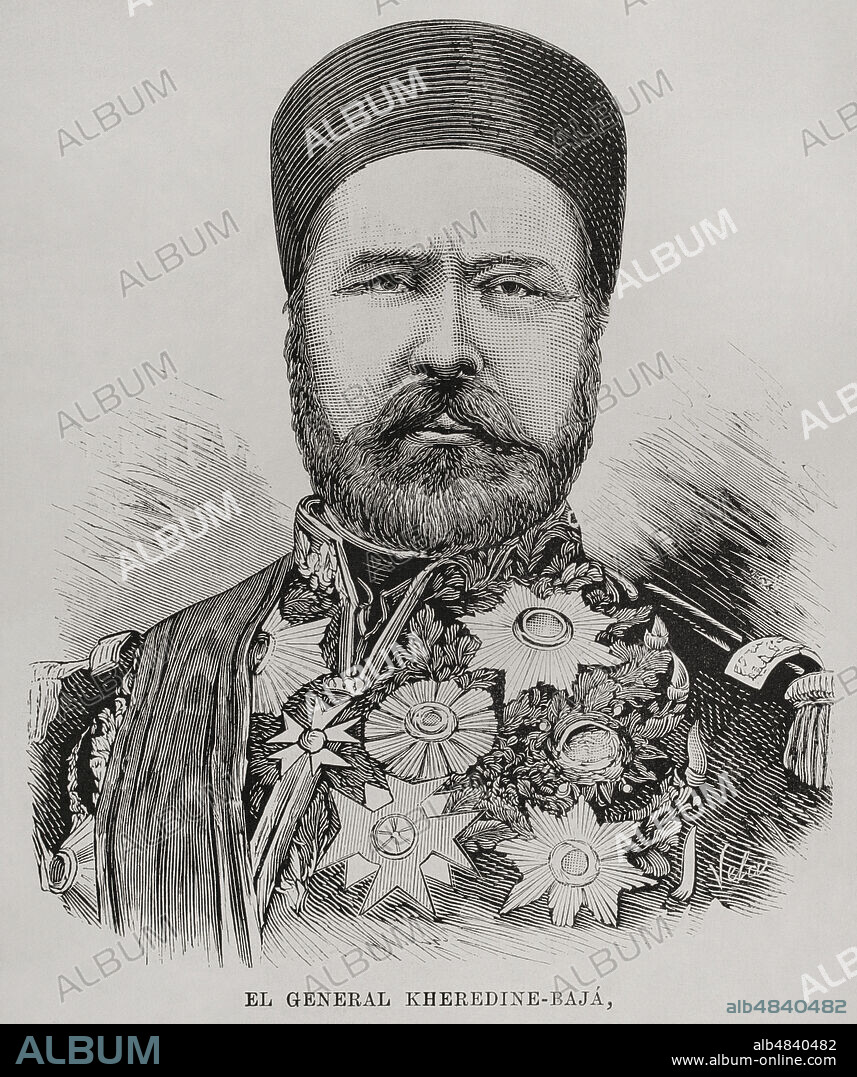This grayscale ink and pencil drawing depicts a well-decorated soldier named El General Carradine Baja. He wears a tight woven hat that resembles a turban or pillbox hat, and his face is adorned with a long mustache and a short, cropped beard, giving him a regal and serious expression. His uniform is adorned with numerous medals and decorations on his chest and shoulders, including decorative metals and epaulets, which emphasize his high rank and decorated status. He also wears a sash across his left shoulder. The drawing is on a gray background and is watermarked with the word "album" in varying shades of gray and white. At the bottom, it includes a black section with text in a bluish font that reads "album" along with additional information, "AB-4840482" and the website URL www.album-online.com, which is repeated above in blue font on the gray background. This detailed portrait likely dates back to the 1800s or early 1900s and features a man who appears to be of Indian or Middle Eastern descent.